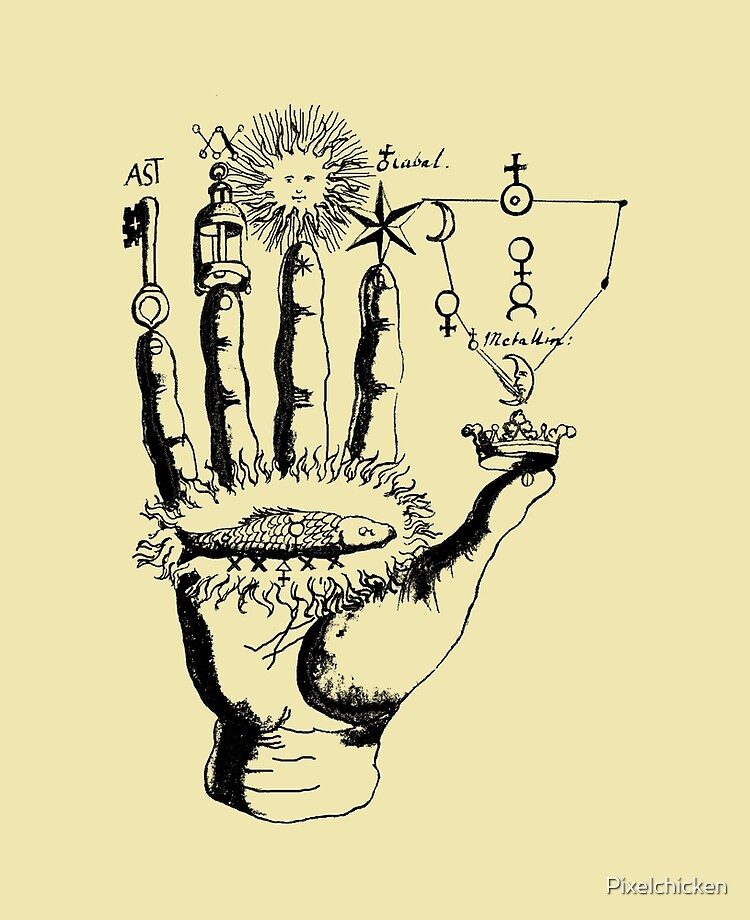The artwork is a detailed black and white pen drawing in the style reminiscent of a Renaissance piece, akin to something Da Vinci might have created. The background of the image is a solid yellow color with the text "Pixel Chicken" positioned in the bottom-right corner in a white font bordered in gray. The central subject of the artwork is a highly detailed human hand with all five fingers spread out. 

Above the pinky finger, on the left side of the image, there is a key with the letters "A-S-T" inscribed on it. To the right, the ring finger features a lantern-like object and a W-shaped symbol. The middle finger is adorned with a sun-like object that has a face. The pointer finger features a six-pointed star with some text above it. On the thumb, there is an intricately drawn crown, and just above it, there are additional symbols, including a moon, a female sign, another moon, a crescent moon, an upside-down female sign, and several lines.

Centered in the palm area of the hand is a detailed drawing of a nest and a dead fish. Additionally, there are four X's at the bottom of the artwork within the palm. This Renaissance-styled drawing integrates various symbolic elements on each finger and the palm, creating a complex and intriguing visual narrative.